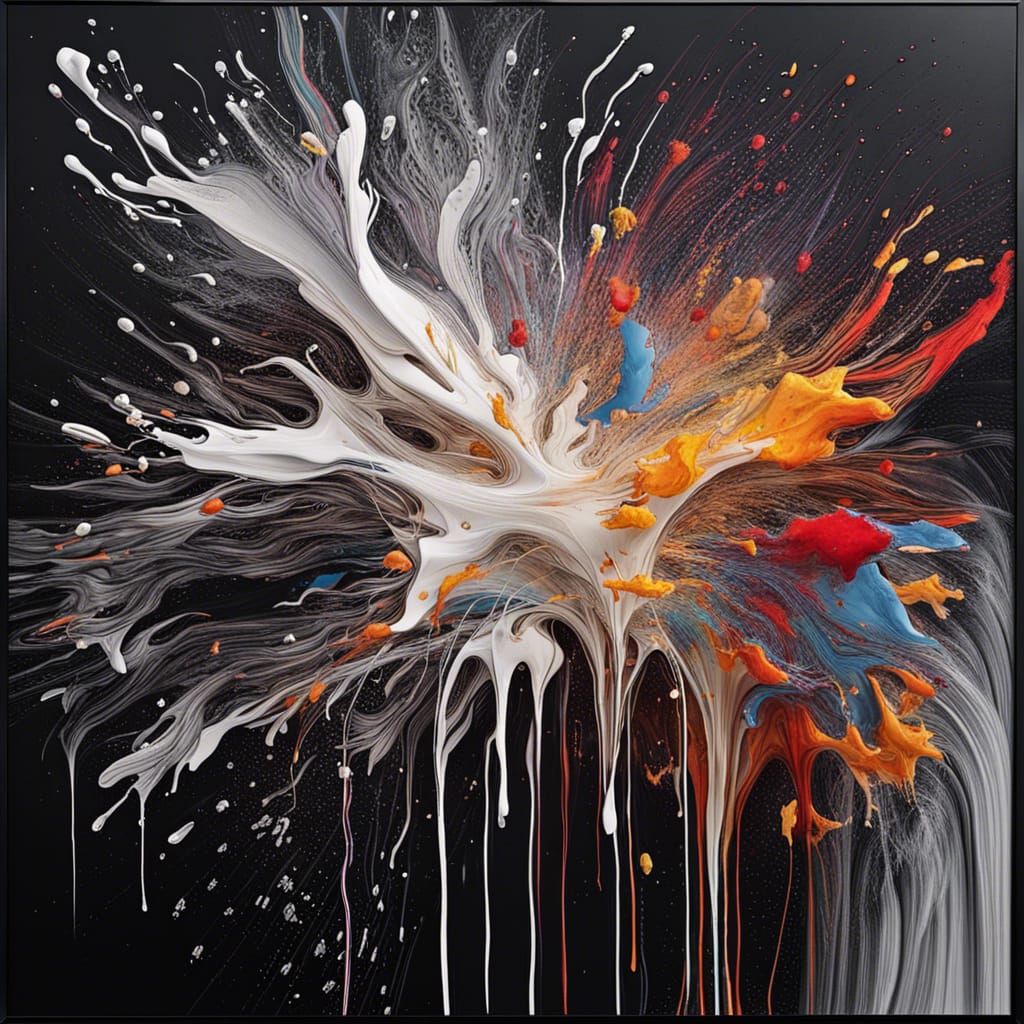The image depicts a square digital painting characterized by an abstract, modernist style against a stark black background. The central focus is an explosion of paint colors that seem to burst outward and then cascade downward. Dominated by white, the vibrant splatters include shades of blue, red, gray, and yellow, creating dynamic, intertwining trails as they descend. This interplay of colors resembles a chaotic, yet meticulous splatter that conveys both the violence of an explosion and the gravity of dripping paint. The painting's black background and subtle frame accentuate the vividness and movement of the colors, giving the impression of the paint either exploding outward or dripping downward, with thin streaks particularly noticeable on the lower right side. The overall effect evokes a sense of energetic motion and fluidity within the confines of a dark space.